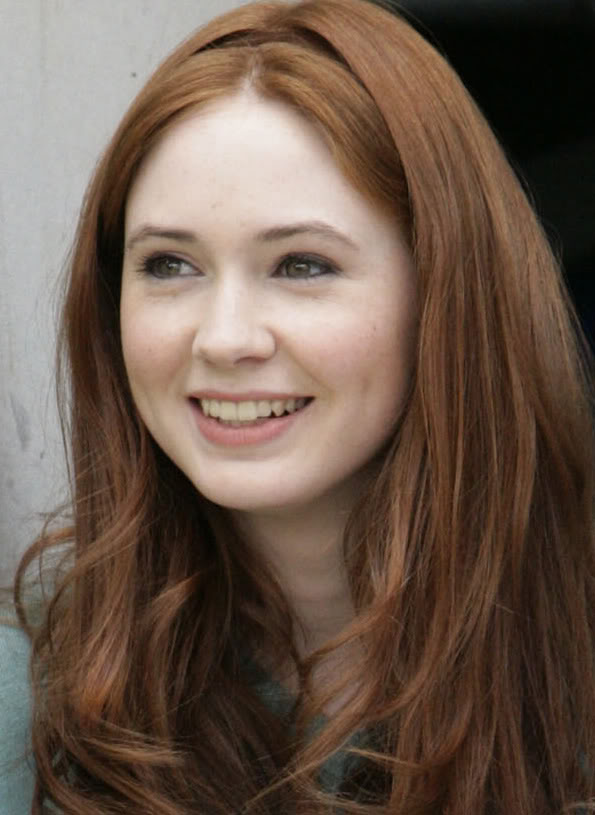This tall rectangular photograph captures a young woman with a familiar, possibly actress-like appearance, seen from her shoulders to the top of her head. She gazes to her left with a slightly tilted head, her smile bright and revealing neatly-aligned top and bottom teeth, with the top slightly overlapping the bottom. Her complexion is very pale with pink undertones, enhanced by light lipstick, giving her a natural look with minimal makeup. Her nose is small and perky above her thinly arched eyebrows and long, possibly artificial, eyelashes. Her thick, long reddish hair is parted in the middle, slightly puffing out on both sides at the top and curling under her chin. She wears a light greenish-gray long-sleeved shirt against a background that features a white wall to the left and a dark area to the right, adding contrast to the image.